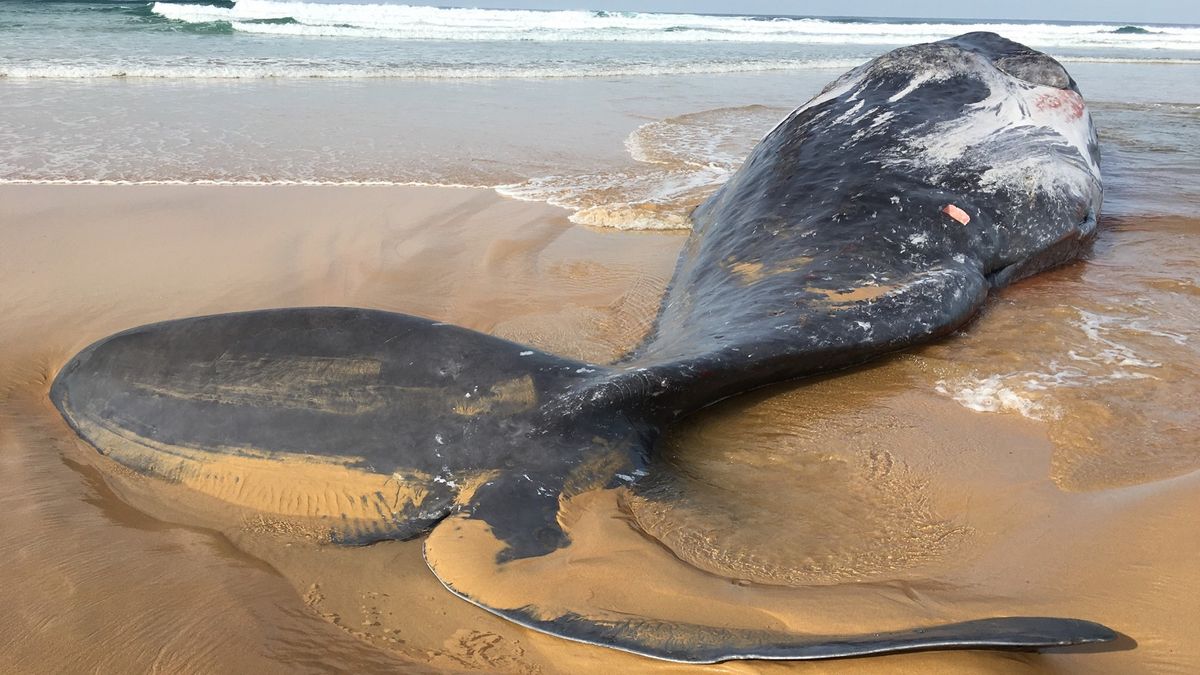This color photograph, taken during the day, depicts a distressing scene of a deceased, beached whale in the center of a sandy beach. The foreground showcases muddy, wet sand of a deep brown hue, with the whale's wide, black body lying slightly turned to its right side. The whale's tail fin is facing towards the camera and is partially covered in the damp sand. Scattered across the body are red blood marks and white scrapings, indicating injuries to its underbelly. White foam and sea salt also speckle parts of the whale. In the distance, gentle rolling waves break, marked by white caps, as they approach the shore.